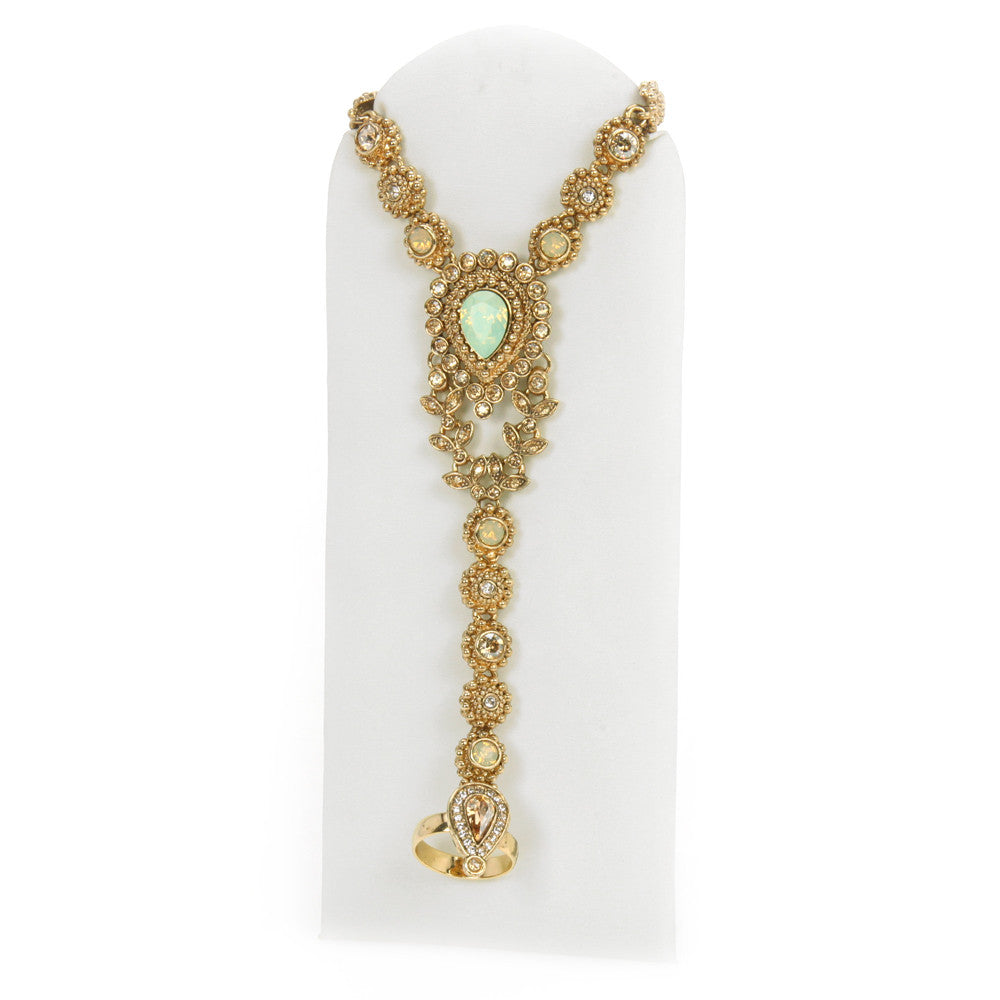The image displays an intricately designed gold necklace showcased on a white velvet or foam jewelry form. The necklace features an elaborate pattern of finely wrought filigree adorned with small gold circles and embedded with clear, crystalline gems. The design is symmetrical, with the gold circles and gemstones creating a repeating motif down both sides. At the center of the necklace, there's a prominent, pale green gem, possibly a semi-precious stone like an opal or a light-colored gemstone. This central gem is surrounded by smaller circular gems and gold circles, forming a leaf-like pattern that extends further down. The necklace culminates in a long, hanging pendant, which appears to terminate in a small ring. The overall effect is one of elegance and intricate detail, making it a standout, uniquely designed piece of decorative jewelry.